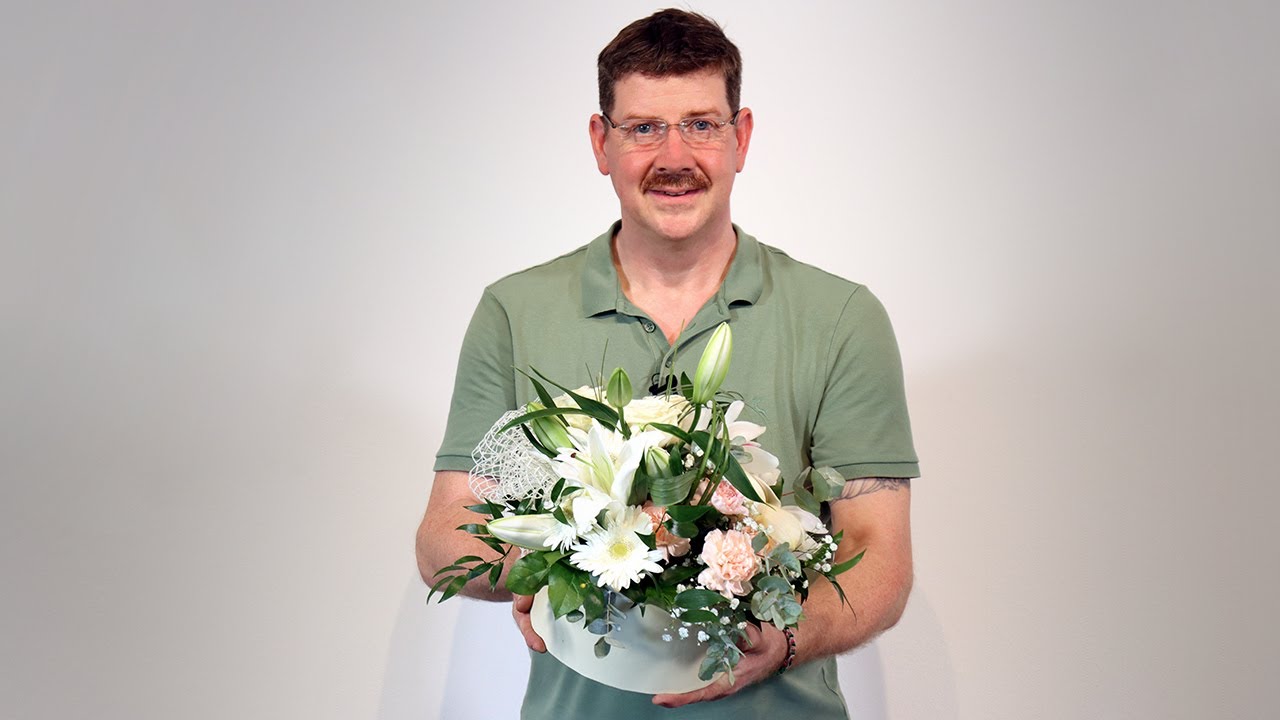In this photo, a man is holding a vibrant floral arrangement presented in a white bowl-like dish with a round plate at the bottom. The bouquet includes a mix of flowers such as daisies, lilies, carnations, eucalyptus, baby's breath, and some unopened white bulbs, all surrounded by a variety of dark green leaves. A white flower with a yellow center blooms prominently at the bottom left, while a pink coiled flower, likely a peony, stands out on the right. Adding to the arrangement is a net-like decorative element on the left side. The man, with very short reddish-brown hair and a thick mustache, is gazing directly at the camera through small-lensed, square-framed glasses. He has an olive green polo shirt with the top button undone, revealing the top of his chest. His right arm displays the bottom part of a tattoo wrapping around his forearm or bicep just below the sleeve, and he wears a dark brown watch on his left wrist. The background features a white to light gray gradient with bluish-gray shadows cast on the wall, indicating he is lit centrally in the frame. The overall impression is of a carefully composed, almost stock-photo-like quality image.